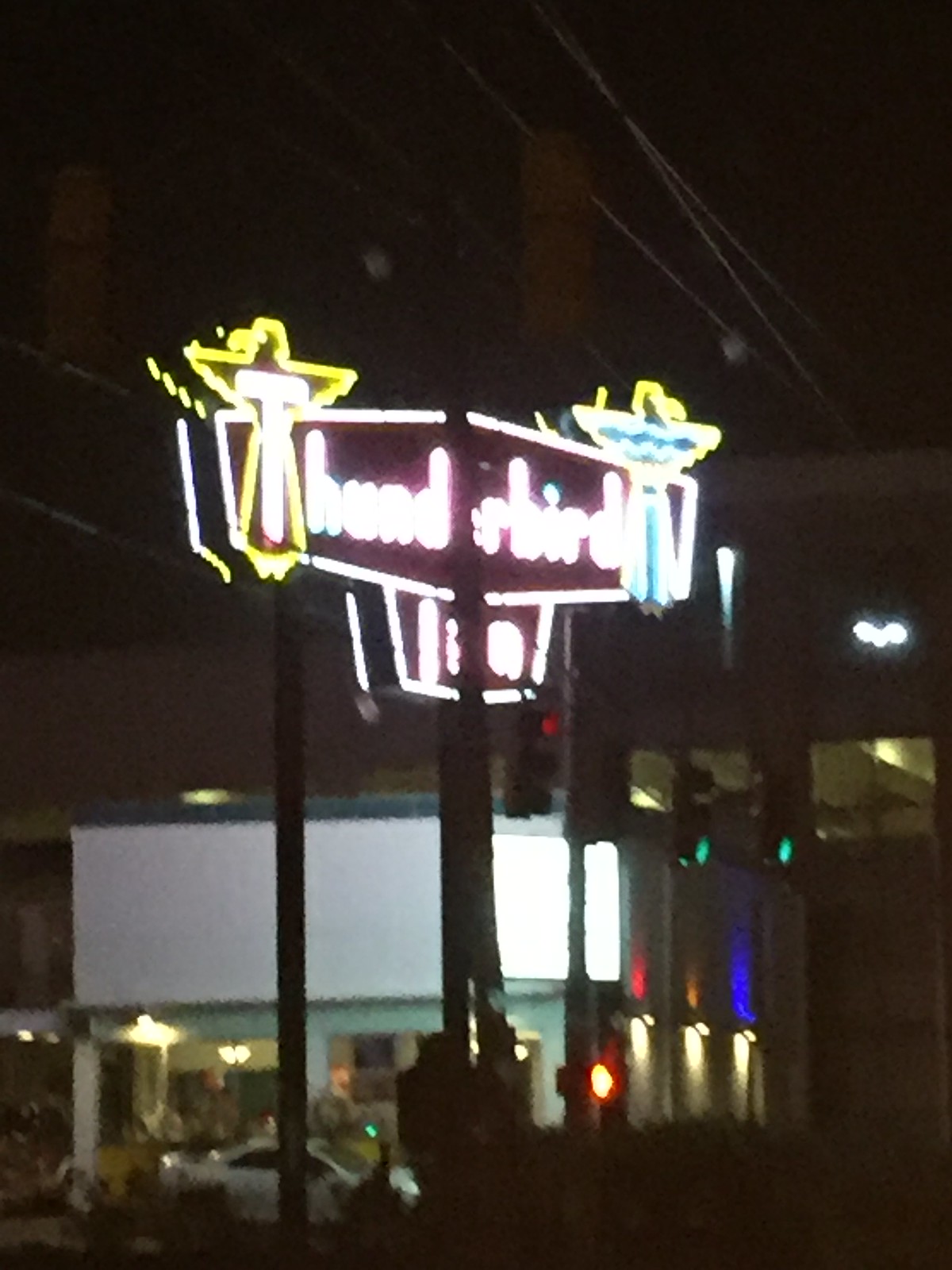This photograph, taken at night in an urban setting, features an out-of-focus neon sign as its main subject. The backdrop reveals a vibrant cityscape illuminated by a myriad of neon and street lights. Central to the image is a neon light sign mounted on a vertical pole, extending horizontally on both sides. The sign prominently displays the word "THUNDERBIRD" at the top in capital letters. The 'T' in "Thunderbird" is distinctly highlighted in white and outlined with a yellow thunderbird symbol. At the opposite end of the sign, there appears to be another thunderbird symbol filled with blue neon light. The colors in the sign include shades of blue, pink, white, and yellow, casting a colorful glow. Despite the intriguing composition, the photograph suffers from significant blurriness, obscuring the details and making the view indistinct.